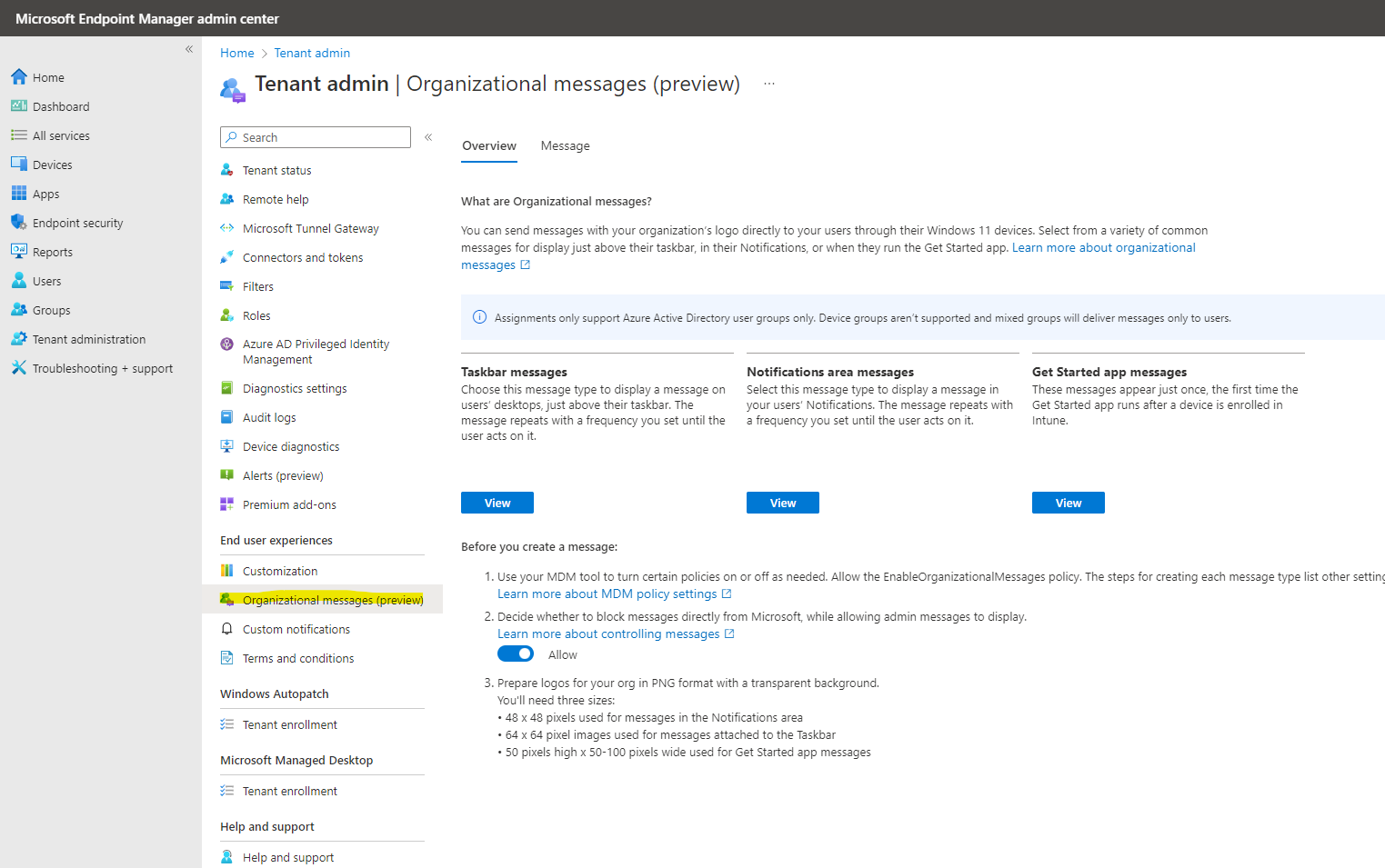The image depicts the Microsoft Endpoint Manager Admin Center interface. At the top, there's a black header with the platform's name. On the left side, a vertical blue navigation menu lists options such as Home, Dashboard, All Services, and Apps. 

Dominating the center is a large white workspace area. At the top of this section, you'll find tabs labeled 'Home' and 'Tenant Admin.' Below these tabs, there are two icons: a small blue bag and a small purple box, accompanied by the text 'Tenant Admin Organizational Messages Preview.'

A search box sits prominently beneath this header. The central portion of the workspace is populated with multiple items, one of which is outlined in yellow, making it stand out. On the right side, the word 'Overview' is underlined in blue, next to 'Message,' indicating a focus on message management.

Further down, there's a blue box with a clock icon in the corner, followed by options for 'Taskbar Messages,' 'Notifications,' 'Message,' and 'Get Started App Messages,' each accompanied by a blue 'View' button. Instructions for creating a message appear below these options, complete with a blue toggle switch under a step labeled 'Number 2.'